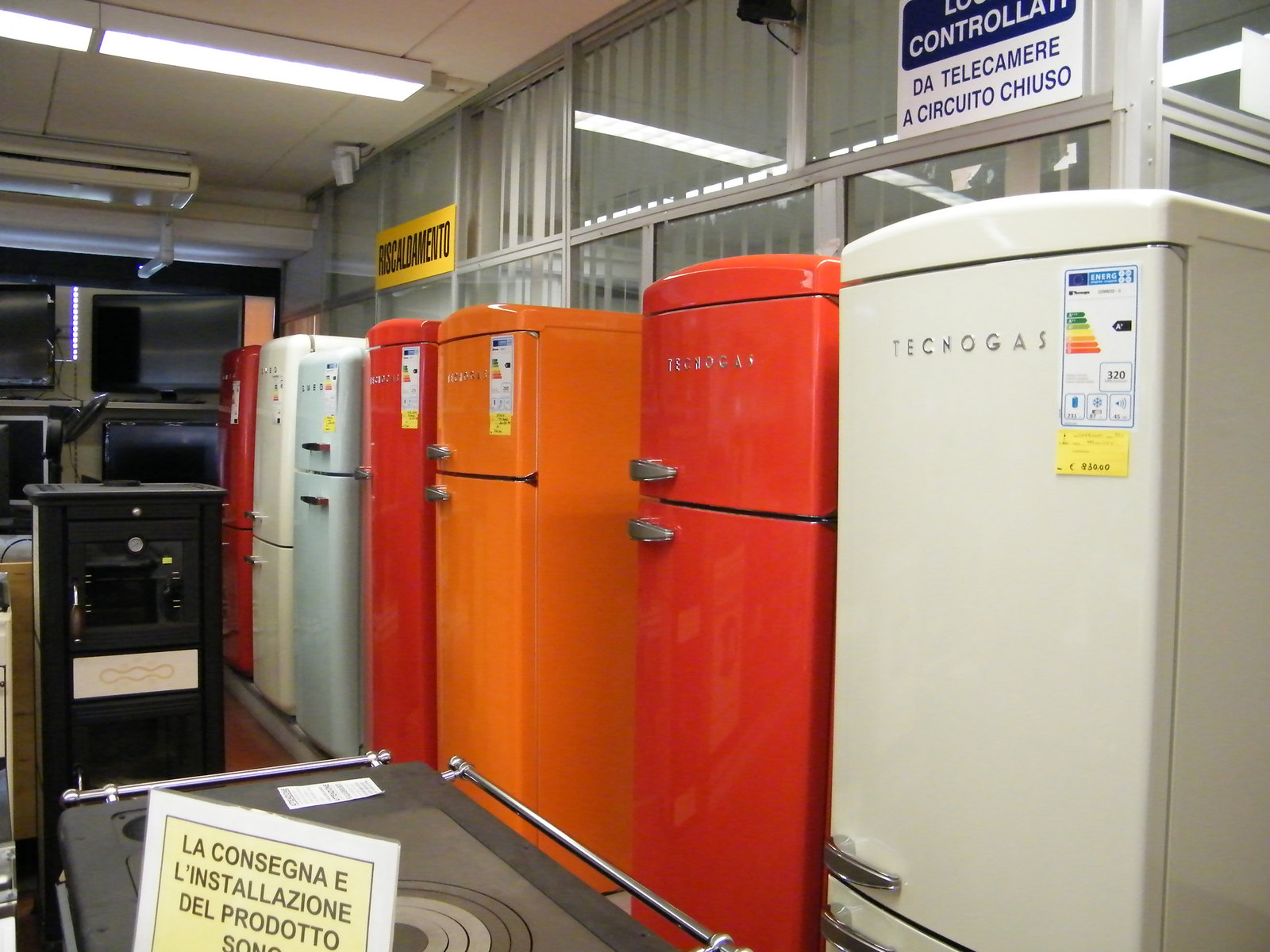The image depicts the interior of an appliance store predominantly featuring older model refrigerators lined up in a row. The store has Spanish signage, suggesting it is located in a Spanish-speaking country. The refrigerators display a mix of colors including white, red, orange, and a very pale blue. Each fridge bears the brand name Tecnogas, along with an energy efficiency rating emblem. Visible in the background is a glass wall with silver metal framing and white curtains. There is also a row of black televisions mounted on a shelf. The store contains other appliances as well, such as stoves and what appears to be a disc player with a sign in black and white. Additionally, one of the stoves features a sign that includes the phrase "La consigna e installacion del produto." The overall setting gives the impression of a vintage or second-hand appliance store, characterized by its drop ceiling with fluorescent lighting and older style refrigerators with large silver handles.